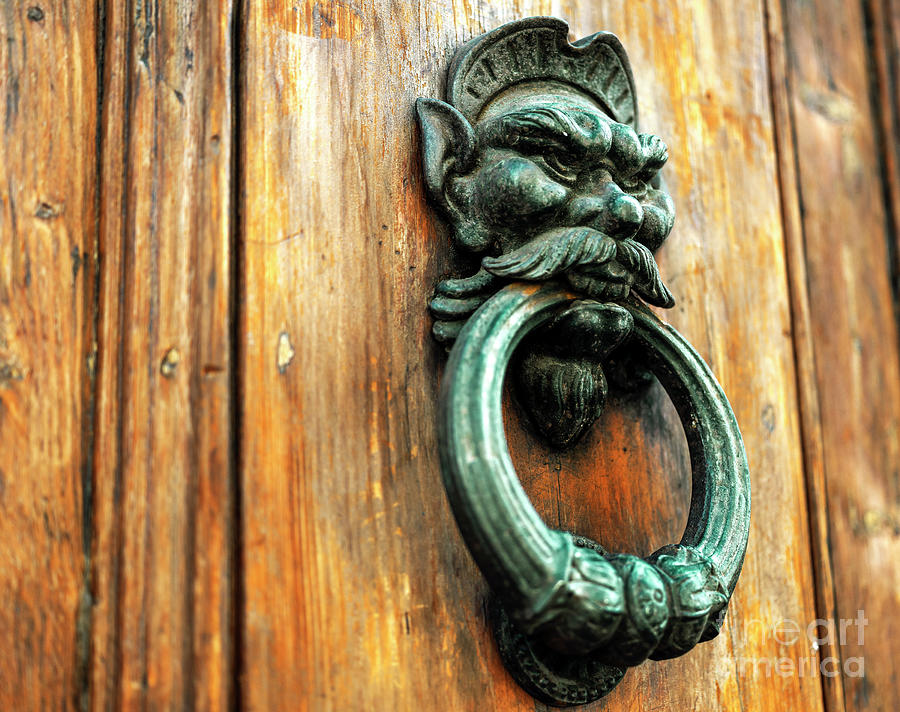The photograph shows a weathered, wooden door adorned with a brass door knocker, covered in a green patina, giving it a seafoam green hue. The door itself has deep grooves and chips, suggesting it's very old and well-worn, with a reflective sheen from a lacquer finish. The knocker features a character that resembles a monstrous creature or gargoyle with a mean expression, pointy ears, large eyebrows, and an oversized mustache reminiscent of the Monopoly man. The creature's mouth holds a heavy, round knocker ring, detailed with beading at the bottom, designed for knocking. A partially visible watermark in the bottom right corner indicates that the image is from a stock photo site. The door is situated outdoors, as suggested by the visible bit of sky in the reflection.